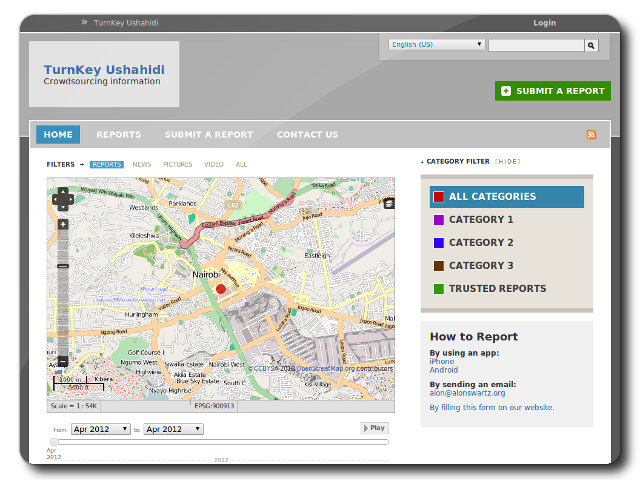**Caption:** 

A detailed screenshot of a website displayed on a tablet in landscape orientation, with rounded corners. The interface features a dark grey bar at the top with a login button on the right. The top left displays "Turnkey Ushahidi" in white text. Below the dark bar, there's a wide light grey band containing a white rectangle with the text "Turnkey Ushahidi" in blue, along with the tagline "crowdsourcing information" underneath. The light grey band includes a drop-down menu set to "English US," a search bar with a magnifying glass icon, and a green rectangular button labeled "SUBMIT A REPORT" in white, all caps.

The bottom half of the screen features a map, with a prominent red dot marking Nairobi, Kenya. A vertical sliding bar on the right side offers zoom control, while a directional navigation cross allows movement in all cardinal directions. A scale in kilometers is located at the bottom left of the map.

Across the top of the map, a horizontal menu includes options: Home (highlighted in blue), Reports, Submit a Report, and Contact Us. To the right of the map, a section labeled "Category Filters (Hides)" allows users to filter reports by various categories: All Categories (red), Category 1 (purple), Category 2 (blue), Category 3 (brown), and Trusted Reports (green).

Below the category filters, there is a text box with instructions on reporting methods. Users can report via an app (with clickable links for iPhone and Android), by sending an email (clickable link provided), or by filling out a form on the website (also a clickable link). The clickable parts are highlighted in blue.